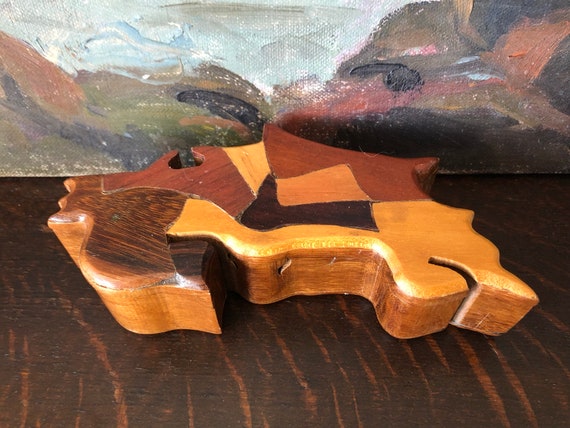The photograph appears to be taken in an artist's studio, showcasing a smooth, curvy, and abstract wooden sculpture made from a collage of various wood pieces in different shades and textures of brown, ranging from light tan to dark. The wood has been cut into intricate shapes, then glued back together to form a unique, possibly face-like design. The sculpture rests on a dark brown wooden floor that's scratched and shows signs of age. Behind the sculpture, the lower part of an oil painting is visible, with a palette of dull, earthy tones—browns, reds, and blues—indicating an abstract theme with subdued brush strokes. The scene is captured in a slightly blurry photograph, making finer details challenging to discern.